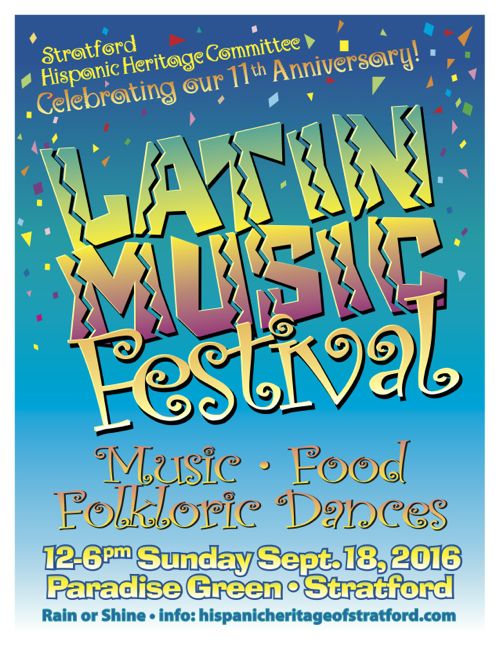Flyer for Stratford Hispanic Heritage Community's Latin Music Festival

Experience the vibrant celebration of the Latin Music Festival presented by the Stratford Hispanic Heritage Community. Set against a gradient blue background that transitions from deep blue at the top to white at the bottom, the flyer immediately catches the eye with its festive design.

At the heart of the flyer, the bold and colorful title "Latin Music" stands out, featuring a dynamic zigzag break within each letter. This vibrant gradient text shifts seamlessly from green at the top, through yellow, and culminates in red at the bottom. Below it, the word "Festival" is displayed in a lively, party-themed font with playful curls, also rendered in bright yellow.

At the very top of the flyer, "Stratford Hispanic Heritage Community" is written in a similar, cheerful yellow font, echoing the playful style of the word "Festival." Just below this, the phrase "Celebrating our 11th Anniversary" adds a note of special significance to this year's event.

Adding to the festive atmosphere, the background is adorned with a confetti pattern, evoking a sense of joy and celebration. The bottom section of the flyer details the array of activities to expect at the festival, including live music, delicious food, and traditional folkloric dances.